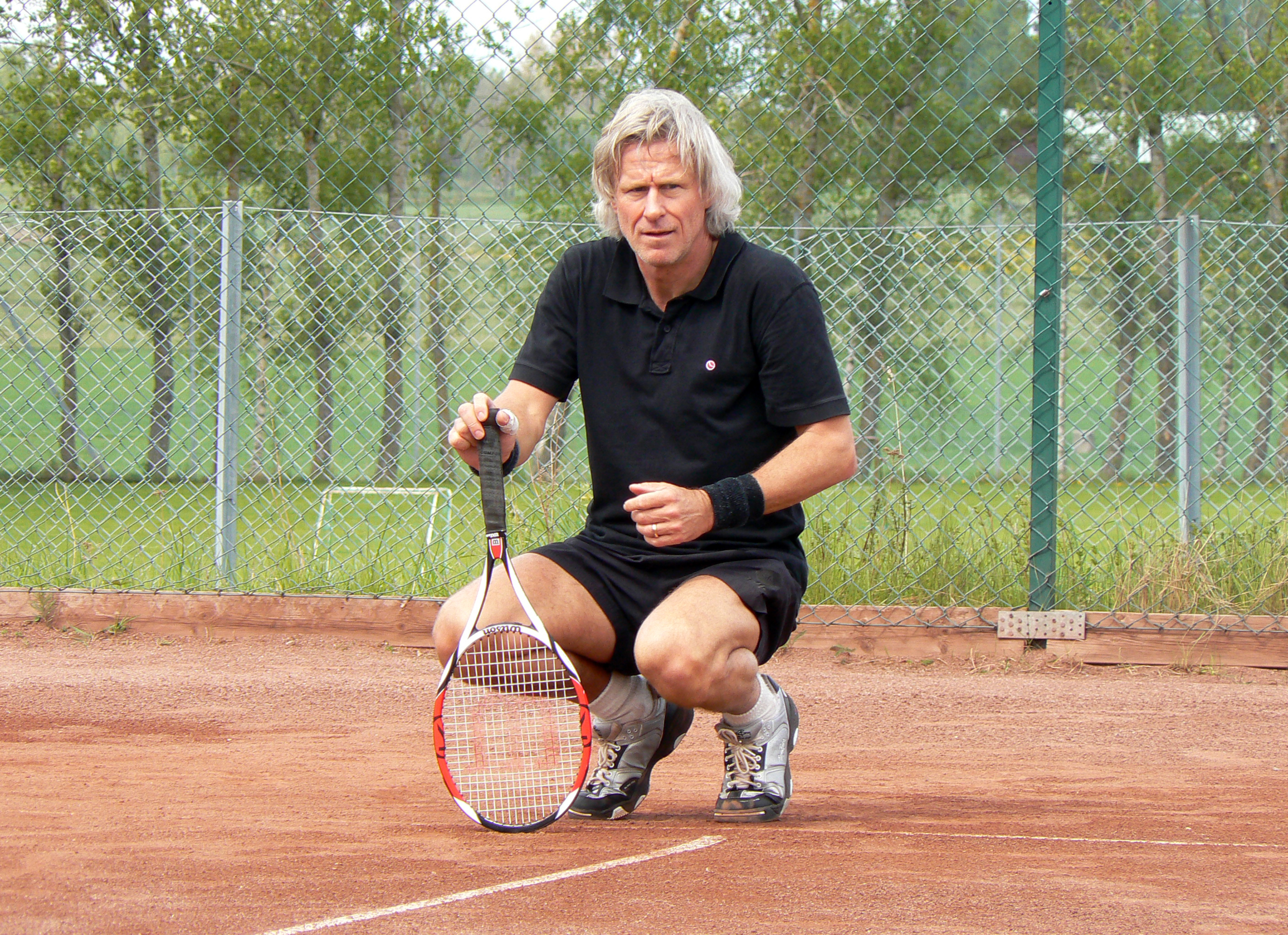In this outdoor photograph, an older man with long white hair is squatting down on a clay tennis court. He is dressed in a black collared short sleeve shirt and black shorts. On his wrist are wristbands, and he wears white and gray shoes with black accents on the soles. In his right hand, he holds a tennis racket, gripping it by its black handle. The racket itself is primarily white with black designs and hints of orange, and features an orange "W" in the center. The tennis court has white chalk lines marking its boundaries. Behind the man, a tall chain link fence can be seen, with another shorter fence visible further back. Beyond these fences, a lush row of green trees and very tall grass extend into the background. On the left side, part of a soccer field with a goal net is just visible, and in the far distance, a building peeks through the foliage.